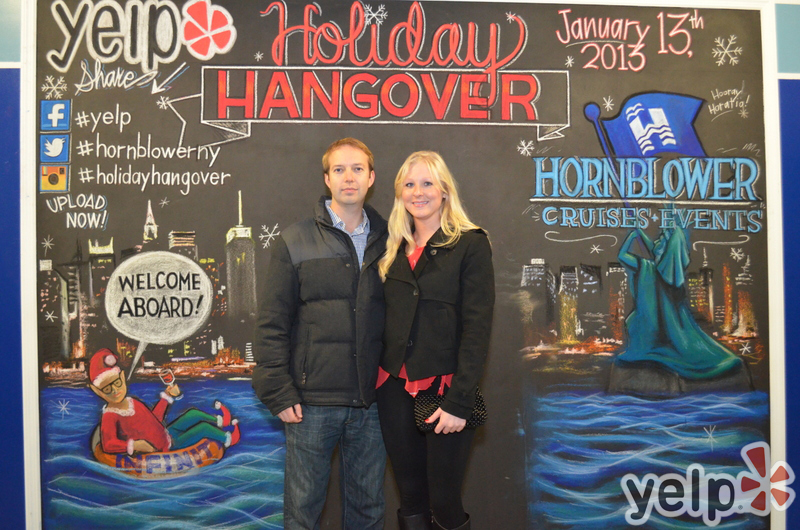The image captures a man and a woman posing together, facing the camera against a detailed backdrop wall. The wall features the slogan "Holiday Hangover" prominently, with "Yelp" in the top left corner and the date "January 13th, 2013" in the top right. The backdrop is adorned with a drawing of a skyline with water, and a festive character on a water tube labeled "Welcome Aboard." The tube has the word "INFINITE" on it. The left side of the image showcases the Facebook logo with the hashtag #Yelp, the Twitter logo with the hashtag #HornblowerNY, and the Instagram logo with the hashtag #HolidayHangover. On the right side, it reads "Hornblower Cruises & Events," with another Yelp logo and wordmark in the bottom right corner. The couple is dressed warmly, with the man in a black jacket, blue shirt, and jeans, while the woman wears a black jacket, red shirt, black leggings, and boots.